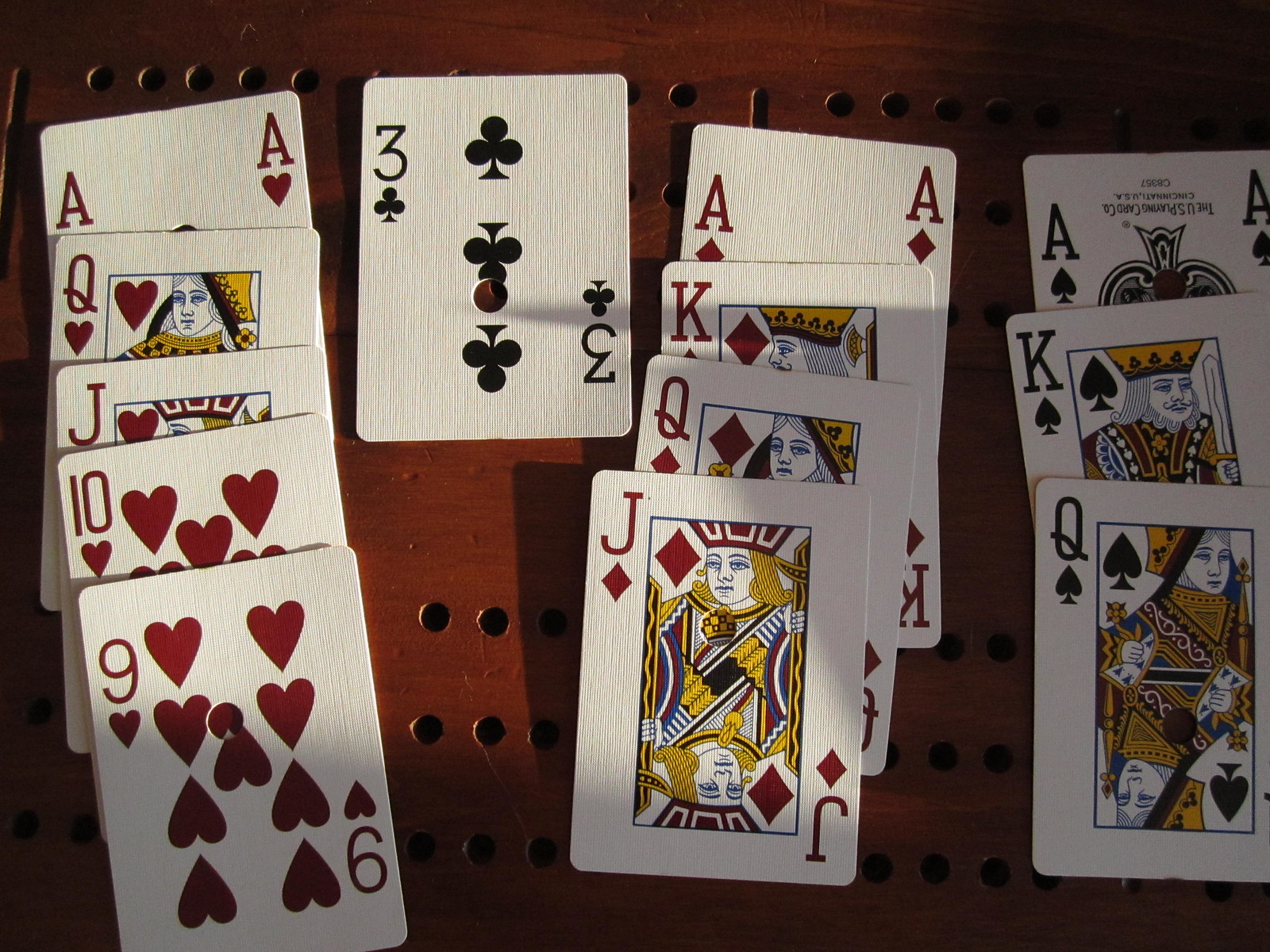The photograph captures a detailed arrangement of playing cards on a wooden table with a distinct dark brown surface punctuated by numerous small round holes of unknown purpose. The cards are positioned as though someone is in the midst of a solitaire game, with four clear columns or stacks visible. The first stack features a sequence of red heart cards, starting with the ace at the top, followed by the queen, jack, ten, and nine of hearts. The second stack consists of a single card, the black three of spades. The third column mirrors the first in its red color scheme, with the ace of diamonds on top, followed by the king, queen, and jack of diamonds. The final stack contains three black spade cards, ordered as the ace, king, and queen of spades. The lighting appears to originate from the upper left corner of the image, casting shadows that obscure portions of the lower right cards. Notably, some of the playing cards have holes punched through their centers, adding an additional layer of visual intrigue to the scene.